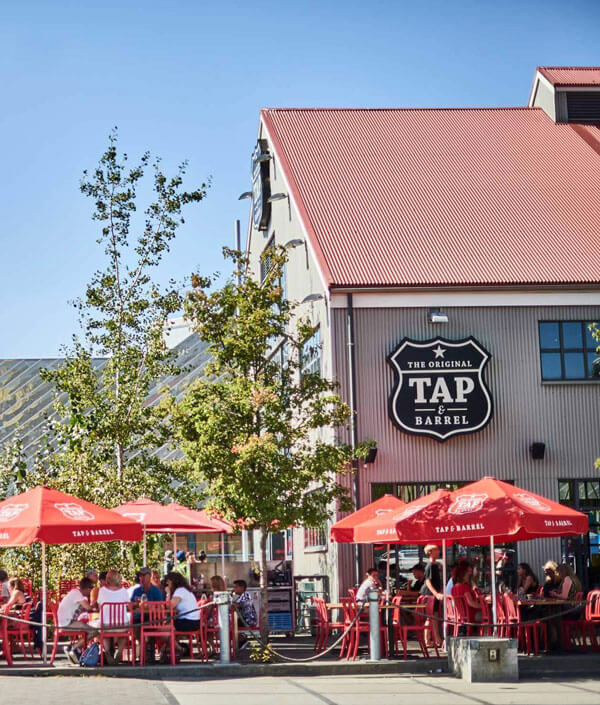In the image, there is an outdoor setting featuring a restaurant called "The Original Tap and Barrel." The establishment is a two-story, large barn-style building with an orange angled roof and panel siding. The scene is set under a clear blue sky, indicating a sunny day in the middle of the day. 

At the bottom of the image, stretching across its width, there is pavement with red seating and parasol umbrellas adorned in white text. Groups of people, predominantly white, are seated under these red parasols, eating and drinking while enjoying their time. Some tables are surrounded by red chairs, and a protective banister lines the sidewalk side of the outdoor seating area.

To the right of the image stands the building with a large badge-shaped sign that reads "The Original Tap and Barrel" in white letters. Light fixtures dot the side of the building. Towards the background, two trees are visible on the left-hand side, adding some greenery to the scene. The top left of the image reveals the blue sky, giving an open and airy ambiance to the restaurant's outdoor dining area.